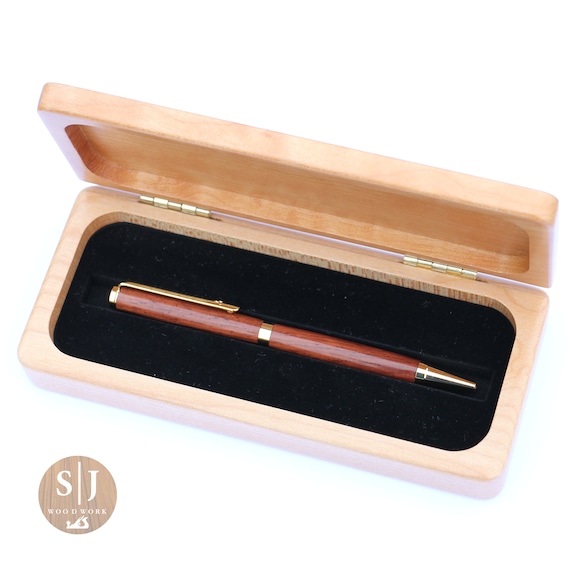This is a detailed close-up photograph of a custom wooden pen housed inside a polished wooden case. The pen, crafted from a dark brown wood with a rich grain pattern, features polished brass accents: a clip at the top, a ring in the center, and a tapered tip. The pen rests in a black felt-lined depression within the case, securing it snugly. The wooden case, made from a light, blonde maple-like wood, is smooth and has rounded corners. It opens via two brushed brass hinges resembling gold, providing a luxurious touch. In the lower left corner of the case, there is a circular logo with a blonde wood-like background, featuring the letters "S" and "J" in white, separated by a line, and the words "Woodwork" printed underneath.